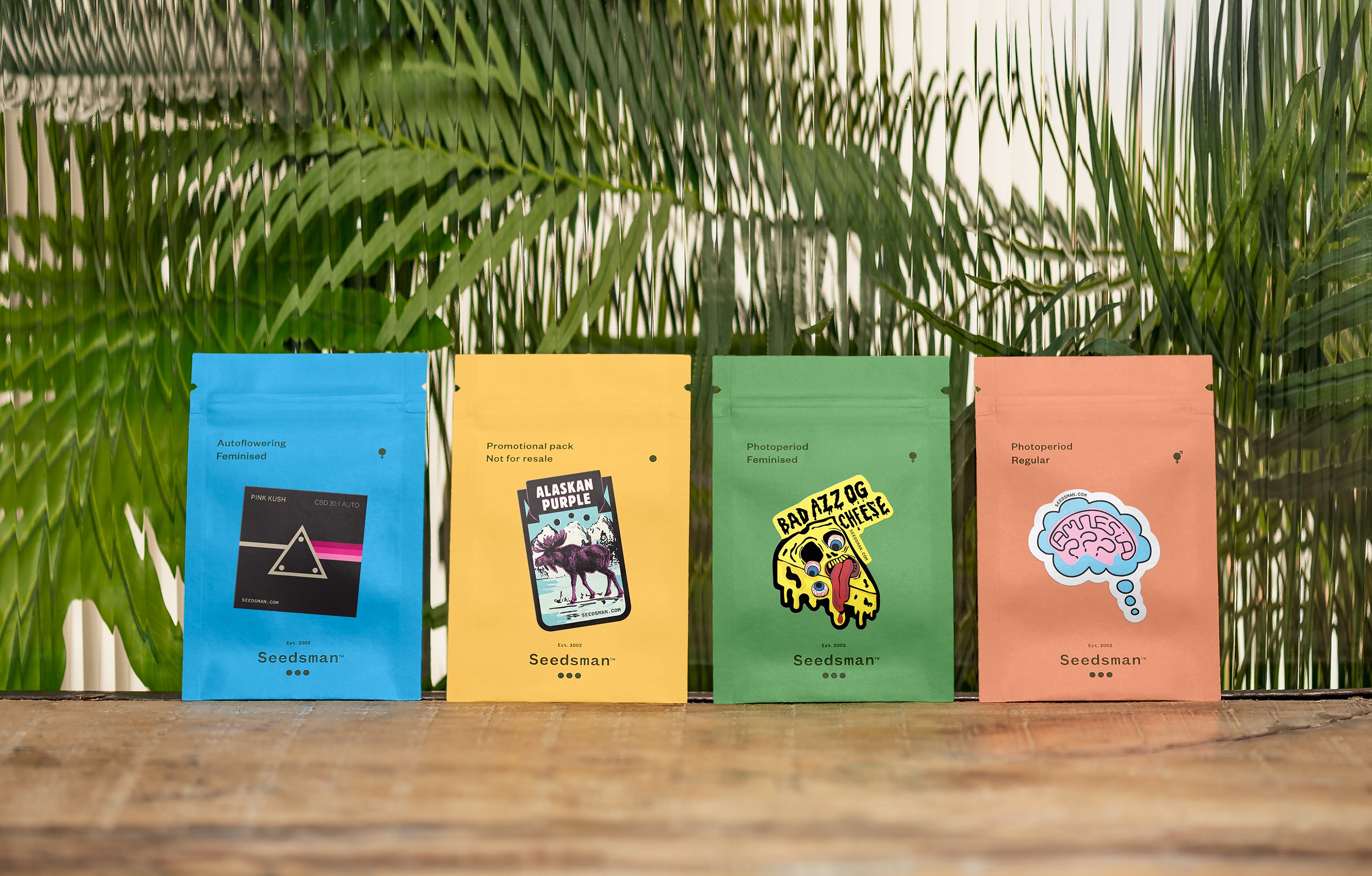The photograph is a rectangular image, measuring approximately six inches wide and four inches high. It depicts a scene with a brown wooden tabletop, placed about three-quarters of an inch up from the bottom edge. Sitting on the tabletop are four colorful, sealed bags arranged from left to right: blue, yellow, green, and coral pink. Each bag features distinct labeling and branding.

In the background, above the tabletop, there is a glass pane with vertical waves which distort the view of the palm fronds behind it, making the leaves appear as zigzagged, green lightning bolts. 

Each sealed bag has notches at the top for easy opening and a reclosable zip area. The branding "Seedsman" is printed at the bottom center of each bag, accompanied by specific details and imagery unique to each package. From left to right, the bags are labeled as follows:

1. Blue Bag: "Auto-Flowering Feminized," featuring "Pink Kush" in the center.
2. Yellow Bag: "Promotional Pack Not for Resale," featuring "Alaskan Purple" and an image of a moose.
3. Green Bag: "Photo Period Feminized," featuring "Badass OG Cheese."
4. Coral Pink Bag: "Photo Period Regular," featuring an image of a brain.

The clear details and vivid colors suggest that these are upscale packages, possibly for seeds. The intricate labeling and distinctive images on each bag indicate a focus on quality and branding, likely intended for a niche market. The entire setup implies the photograph is likely advertising these products.